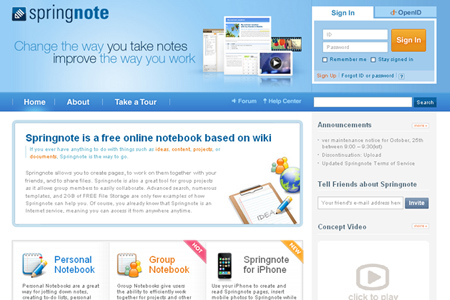In this image, you can see the homepage of an application or website called "Spring Note." The top banner prominently features the tagline, "Change the way you take notes and improve the way you work." Below the banner, there are several images showcasing workflow pages.

To the right side of the screen, the login section is visible, including fields for entering a user ID and password. There is an orange button labeled "Sign In" and next to it, another button labeled "Open ID."

Further down the page, the navigation menu is displayed with links to the Home, About, Take a Tour, Form, and Help Center pages. Additionally, there's a search bar for users to look up specific information. The homepage is currently selected. The text on the homepage presents Spring Note as a free online notebook based on Wiki. It mentions that Spring Note allows users to create pages, collaborate with friends, and share files. The tool is particularly useful for group projects, facilitating easy collaboration among members.

The text continues to describe various features of Spring Note, including advanced search capabilities, a wide range of templates, and 20 gigabytes of free file storage. However, the text becomes blurry towards the end and is difficult to read, though it seems to highlight the benefits and functionalities of the application further. Overall, the webpage provides a comprehensive overview of what Spring Note offers and how it can enhance note-taking and collaboration.